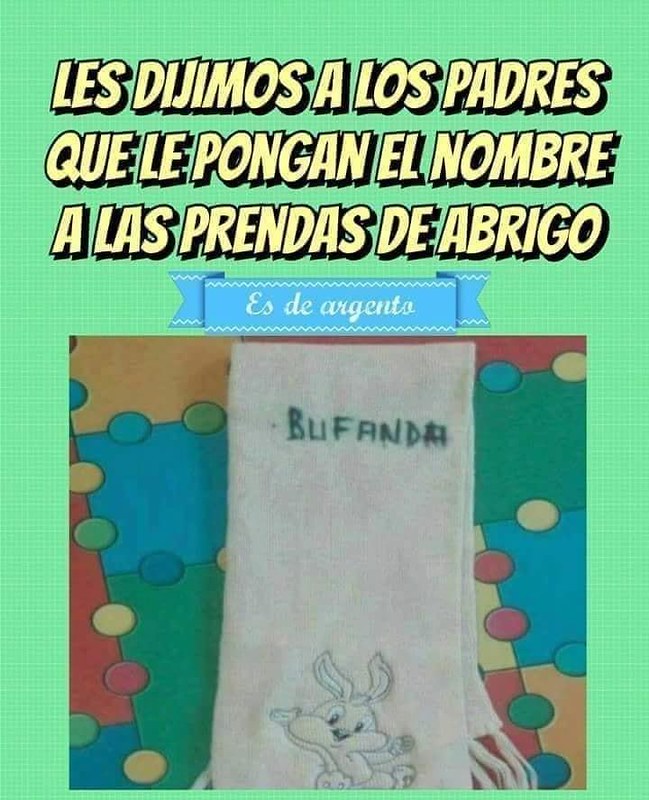This image features an advertisement flyer displayed on a green checkered background. Prominently, at the top, bold yellow text with a black drop shadow reads "Les Digimos a los padres que le pongan el nombre a los prendes de abrigo." Beneath this text, a blue ribbon banner with wavy white lines at the top and bottom showcases the words "Es del Aguenta" in white text. 

Central to the flyer is a photograph of a children's play mat adorned with various colorful patterns, including squares and circles in shades of blue and green. Laying on this mat is a small hand towel or scarf, featuring an image of a Baby Looney Tunes character. The item, inscribed with the word "Bufanda" in black handwritten text, adds a playful and nostalgic touch to the overall composition.